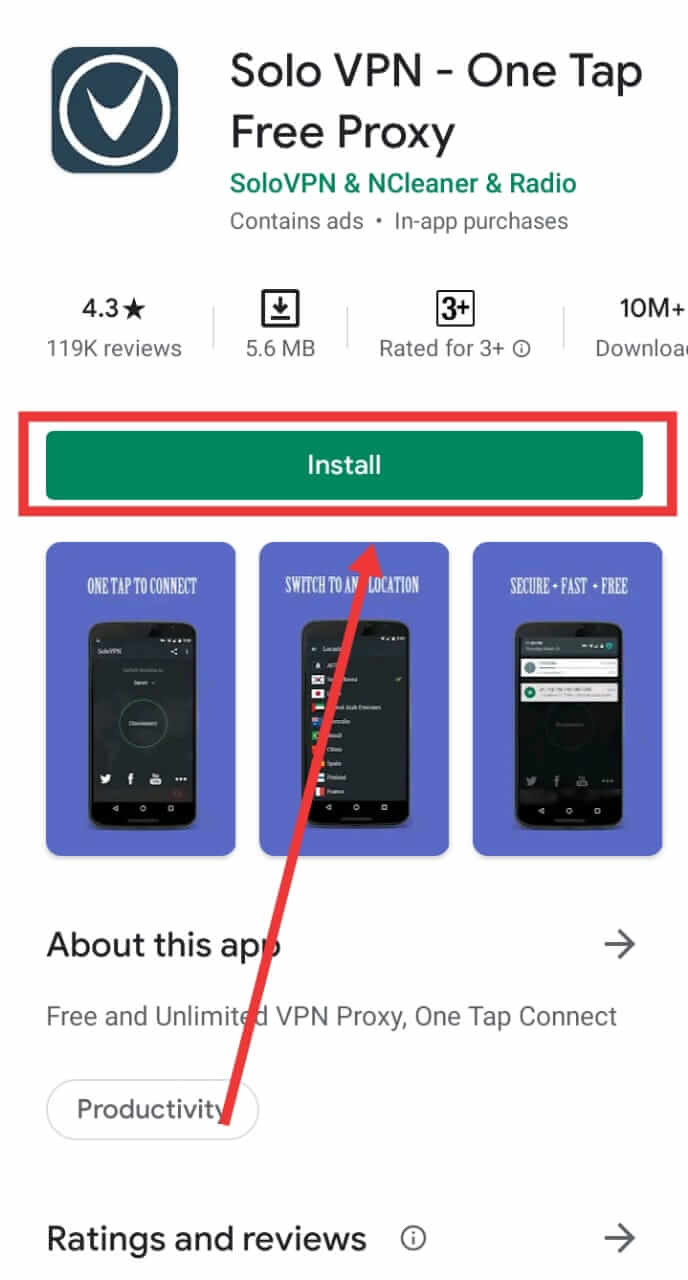At the top left corner of the image, there is a green square featuring a white outlined circle with a thicker V-shaped symbol in the center. Adjacent to this is the text "SOLOVPN" in all capital letters, followed by a dash and the phrase "One-Tap Free Proxy." Below this, in green text, it says "SoloVPN," "NCleaner," and "Radio." Underneath this information, a gray line indicates "Contains ads · In-app purchases." Down the left side, a star symbol next to the text "4.3" is shown, followed by "119K reviews" below it. To the right of this section, there is a square with a downward-pointing arrow and "5.6 MB" underneath. The ratings are indicated as "Rated for 3+," followed by "10M+ downloads."

There is a prominent outlined red rectangle containing a green fill in the center, with the word "Install" placed prominently inside. Below this section, there are three images of cell phones, each housed within long purple rectangles. Further down, the text "About the app" is followed by the word "Productivity" with an arrow pointing right, which is aligned towards the green box with the "Install" button. Finally, at the bottom of the image, the text "Ratings and reviews" is presented with an arrow pointing to the right.